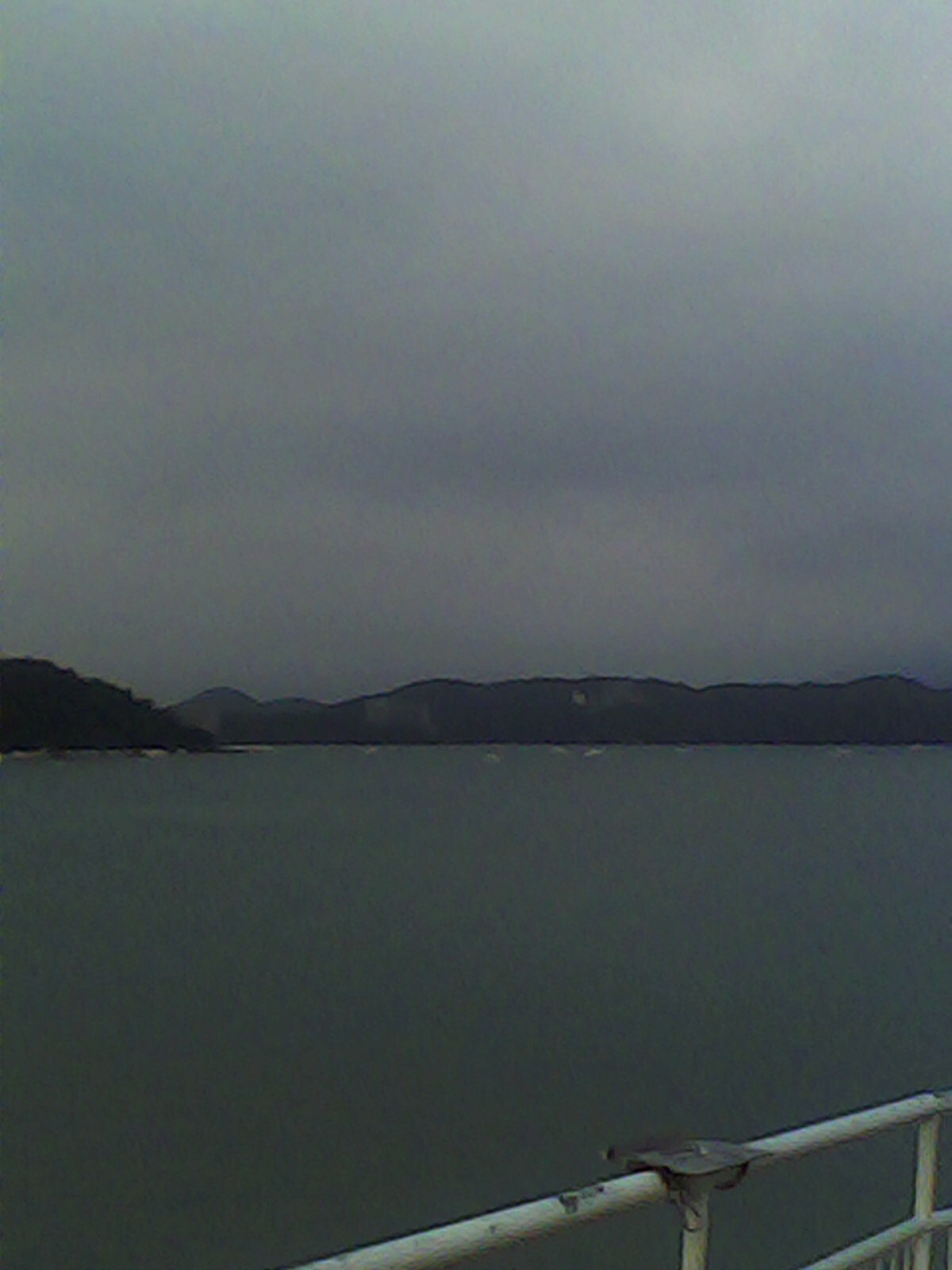The photograph, rectangular in shape and taken outdoors during daylight, captures a dreary, gray day. The sky is completely overcast with a menacing, angry look, enhancing the misty atmosphere of the image. The scene is viewed from an overlook or possibly the side of a ferryboat, evidenced by the presence of a white metal rail in the foreground. This rail stretches across the bottom of the photo, contrasting sharply with the grayish-green, calm body of water it overlooks. In the distance, a small mountain range is visible, contributing to the somber tone of the image. To the left, the water appears to wrap around a small hill or mountain, forming a cove-like area adorned with rough-looking shrubbery and trees. The overall composition is dominated by shades of gray, from the ominous clouds overhead to the still waters below.